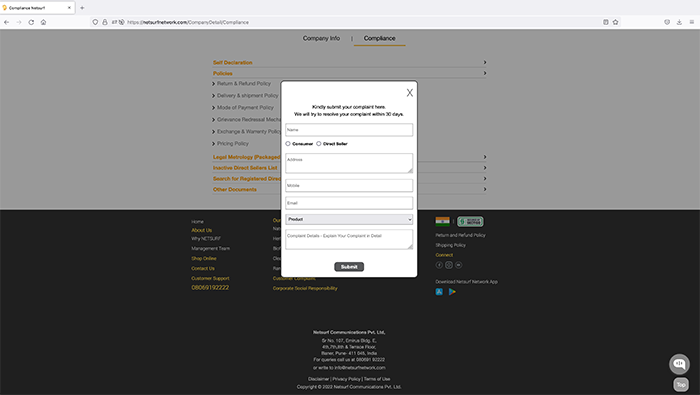A screenshot of a web page displayed on a computer screen features several distinct sections. At the very top, there is a gray navigation bar. Attached to the left of this bar is a white search input field, though the text inside it is not discernible. Below this, a second, slightly lighter gray bar houses several standard browser navigation icons: a left arrow, a right arrow, a reload circle, and a home icon. Adjacent to these icons is another search bar with an address typed in, though it is unreadable. To the right of the search bar, there is a star icon, followed by a left-pointing arrow, a heart icon, a download icon, and a square icon.

Under this navigational layer, the main content area of the webpage is divided horizontally into two sections. The upper half is primarily light gray and includes various company-related links such as "Company Info" and "Compliance," each accompanied by arrows for expansion. The lower half is black, displaying further company details including "About Us," phone numbers, and addresses, although the specific text is too small to read clearly.

In the center of this content area, there is a prominent form requesting the user to fill out fields for their name, address, and email, among other information, with a black "Submit" button at the bottom. This form also features an 'X' at the top corner, allowing users to close it. The overall layout combines shades of gray and black, providing a structured yet monochrome visual experience.